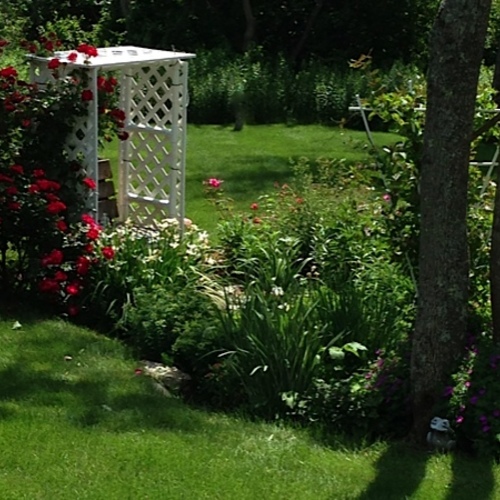This outdoor photograph depicts a picturesque backyard garden. On the right-hand side, two tree trunks frame the scene, one barely visible on the edge, casting distinctive shadows across the well-maintained grass. Between the shadows stands a small, endearing statue of a frog, facing towards the viewer. To the left of the trees, an array of lush green bushes and plants flourish in a meticulously curated garden bed, separated from the grass by a neat layer of mulch. Further left, a quaint wooden chair rests beneath a white trellis, which supports a cascade of deep red roses climbing the left side. The trellis features geometric cutouts, allowing glimpses of the vibrant lawn and various plants behind it. Among the garden's diverse flora are tall grass-like plants, ferns, white and pink flowers, and clusters of irises and foxgloves with their elegant purple blooms. The backdrop reveals a flat, grassy area leading to a shadowy, more untamed section with trees and wild plants, completing this serene garden vista.